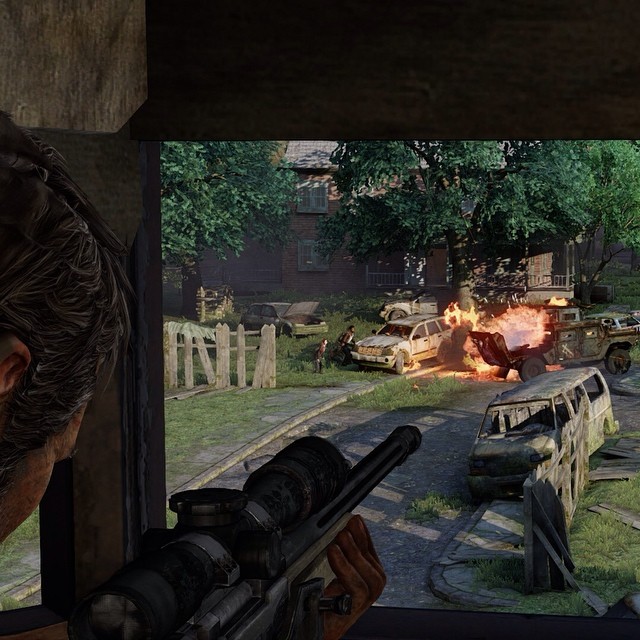A screenshot from a highly realistic first-person shooter game depicts an intense post-apocalyptic scenario. The player, identifiable by the top of his head with short brown hair, is seen wielding a weapon, viewing the desolate landscape through the eyes of his character. The vantage point is from an elevated position, possibly a deer blind or a treehouse, giving a tactical overview.

An overgrown, abandoned road stretches below, cluttered with derelict vehicles. Notably, a Humvee is engulfed in flames, its engine ablaze, with the fire beginning to spread to a nearby tree. The scene is punctuated by burned-out cars and a van, adding to the sense of devastation. 

In the distance, a small red-brown brick apartment building with a gray roof stands, partly obscured by a couple of trees and surrounded by dilapidated, incomplete fencing. The area appears significantly degraded, suggesting a long-abandoned, crisis-stricken neighborhood. Tall grass overgrows the scene, mingling with scattered junked cars, contributing to the overall sense of neglect and ruin. This image captures the chaotic and desolate environment typical of a well-crafted apocalyptic video game setting.